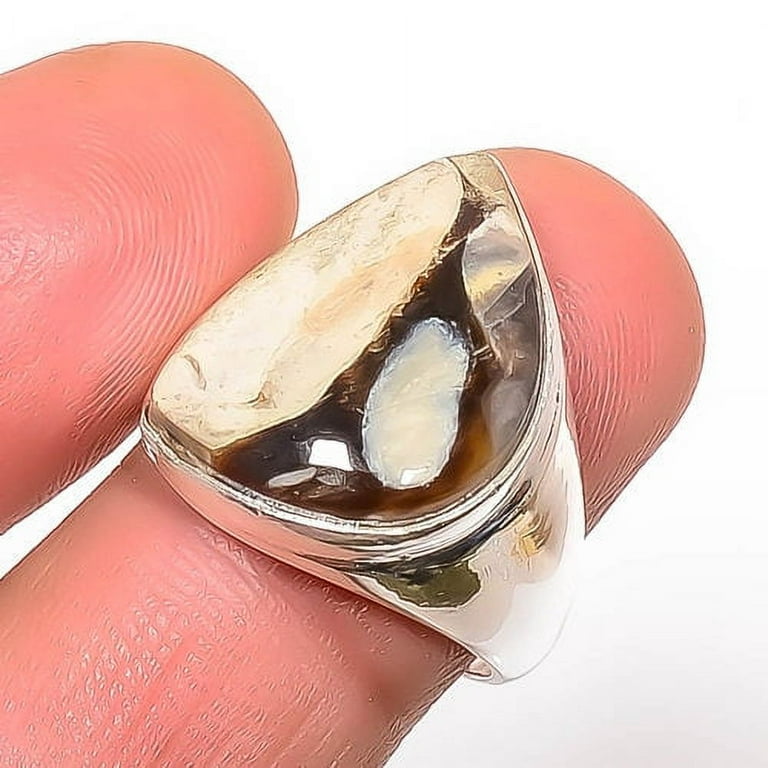The image is an extreme close-up color photograph of two fingers under a very bright, white light, such as fluorescent, halogen, or LED, creating a vivid and detailed view. The focus is primarily on the middle and ring fingers, highlighting their skin's texture, ridges, and fingerprints. The middle finger, which enters from the left and diagonally extends to the right, features a ring on its last digit. The ring is silver, possibly highly polished sterling silver, with a broad, tapered band. It is adorned with a mix of rough-polished stones that resemble gems from geodes, primarily white and yellow, set in a pearlescent black and orange matrix. The ring’s highly reflective surface catches some background light but lacks any distinguishable text or markings. The background is a white and grey gradient, and the lighting emphasizes the details of the fingers and the ring, making the photograph appear exceptionally processed, with a slightly smudgy look due to heavy image processing. There is no nail visible on the fingers, and the entire first knuckle of the middle finger is shown. The image captures the intricate details and textures, down to the reflective chunks and creases along the finger joints.